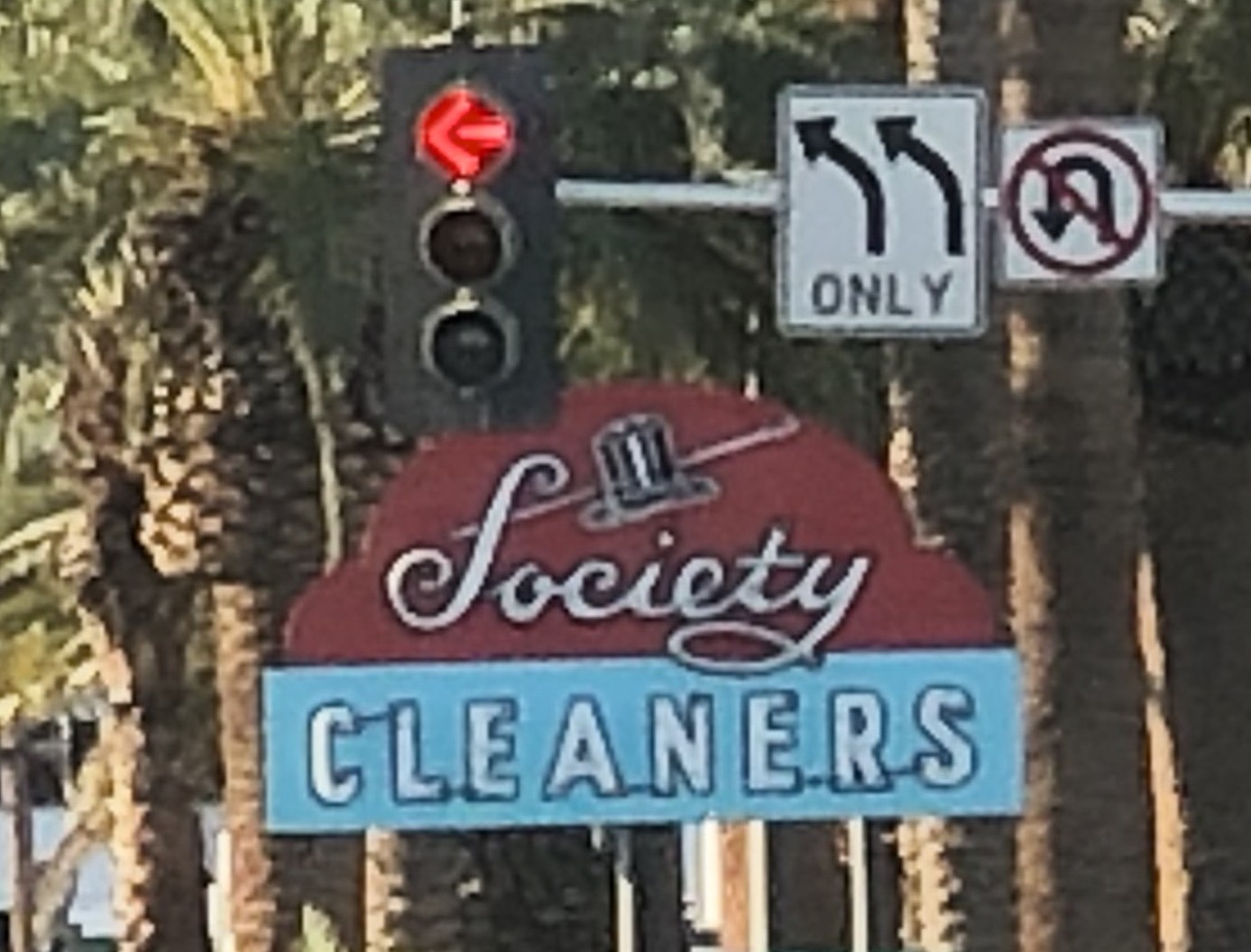The image shows a traffic light mounted on a horizontal pole extending to the right. At the top of the light, there is a red left-turn arrow. Adjacent to the light, a street sign displays two left-turn arrows with the text "ONLY" at the bottom. To the right of this sign, there is another sign indicating "No U-Turn" with a black U arrow crossed out by a red circle. In the background, a sign for "Society Cleaners" is visible, featuring a red background for "Society" and a blue background for "Cleaners," along with an image of a top hat and cane. The entire scene is set against a backdrop of numerous palm trees, characterized by their tall, slender trunks and bushy, green tops. The photo appears to be somewhat blurry, possibly taken from a moving vehicle, indicative of a warm climate due to the presence of the palm trees.